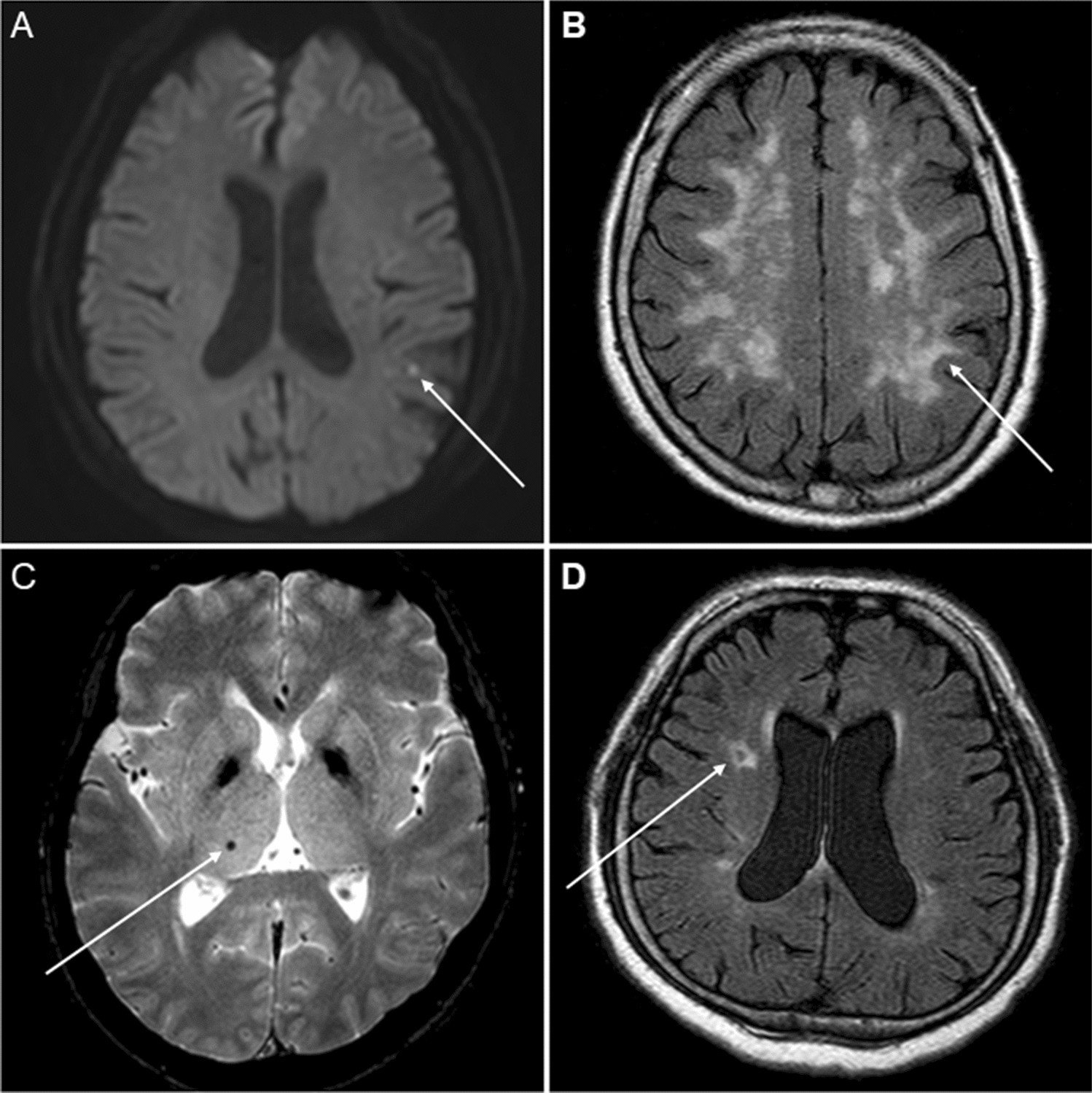This image is a composite of four distinct MRI scans of a brain, arranged in a square grid labeled A through D. Each image highlights different views and characteristics of a brain affected by cancer. 

Image A (top left) is a dark gray scan featuring a white arrow pointing to a small white fleck located in the back right side of the brain, indicating a cancerous tumor. 

Image B (top right) has more white exposure, especially along the border of the skull, with a white arrow pointing to white spots on both sides in the center area of the brain, suggesting multiple tumors.

Image C (bottom left) is a highly fluorescent middle slice of the brain, where a white arrow points to a tiny black dot in the center-left area, indicative of a malignant area.

Image D (bottom right) shows a brain scan with a darker spot surrounded by a white ring in the left front part of the brain, highlighted again by a white arrow, likely pointing to another tumor location.

Each of these scans provides crucial insights into the presence and locations of brain tumors, offering a comprehensive overview of the affected brain.